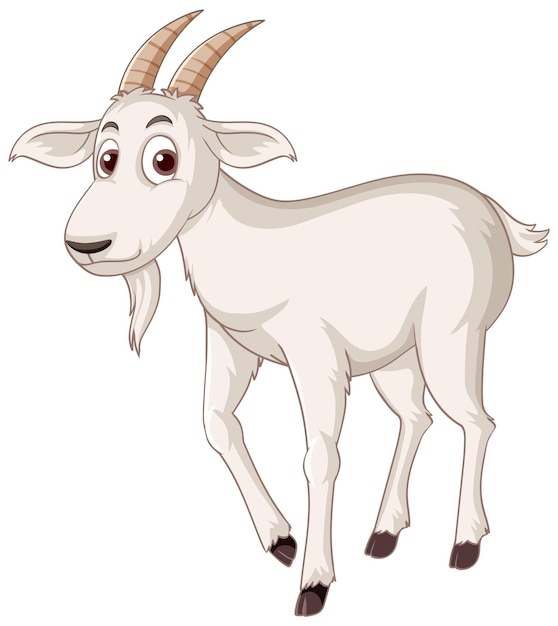The image is a digital cartoon drawing of a white goat standing on a white background. The goat has large, oval, brown eyes and light brown, horn-like structures on top of its head. The goat's nose is a unique green color, and it features matching green eyebrows. The goat is smiling and showcasing a white goatee beneath its chin, which adds to its character. The goat's body includes some dark parts, particularly on the back and belly. It also has black hooves and a small white tail. One of its legs is lifted, giving the impression that it is posing for the picture. The overall style is very cartoonish and simplistic, with some exaggerated features like the goat's curvy, pointy ears and the fanged appearance of its horns.